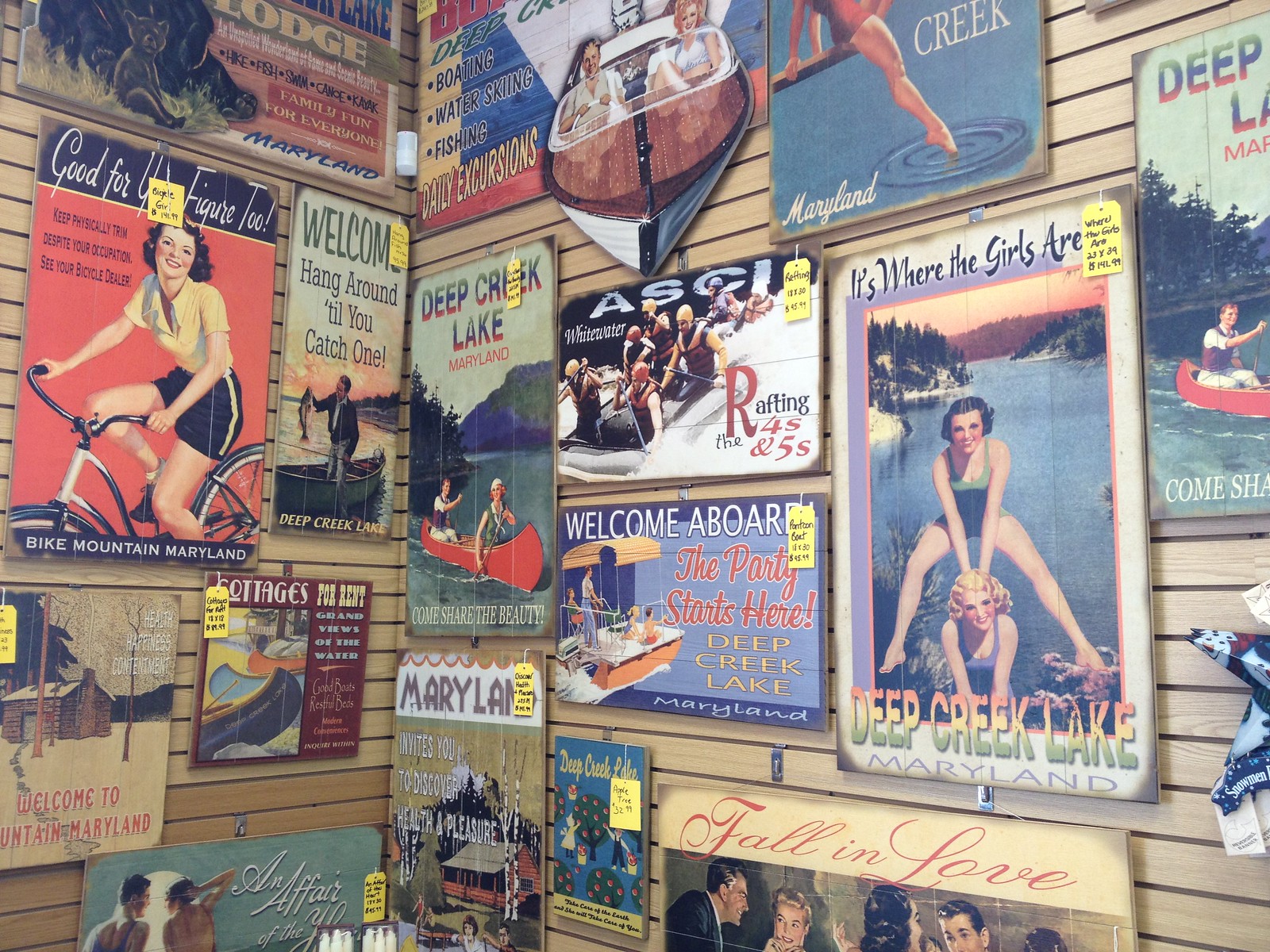The image depicts a vibrant corner of an antique or thrift store showcasing two tan-colored wooden walls adorned with an eclectic array of vintage signs from the 1950s to the 1970s. The signs exude a retro vibe and feature classic cartoon-style illustrations of people engaged in various recreational activities such as cycling, canoeing, boating, and kayaking. Dominantly themed around Deep Creek Lake, Maryland, the signs include cheerful slogans like "Welcome, hang around until you catch one" and "The party starts here." The artwork exhibits a pin-up style, featuring both men and women, with some posters alluding to historical eras like World War I and World War II, evident from the shorter hairstyles of the women. Each sign comes with a small yellow price tag, adding to the nostalgic charm of the display. The collection fills the walls almost entirely, creating a visually dense and engaging composition that invites viewers to explore the storied pasts these signs represent.